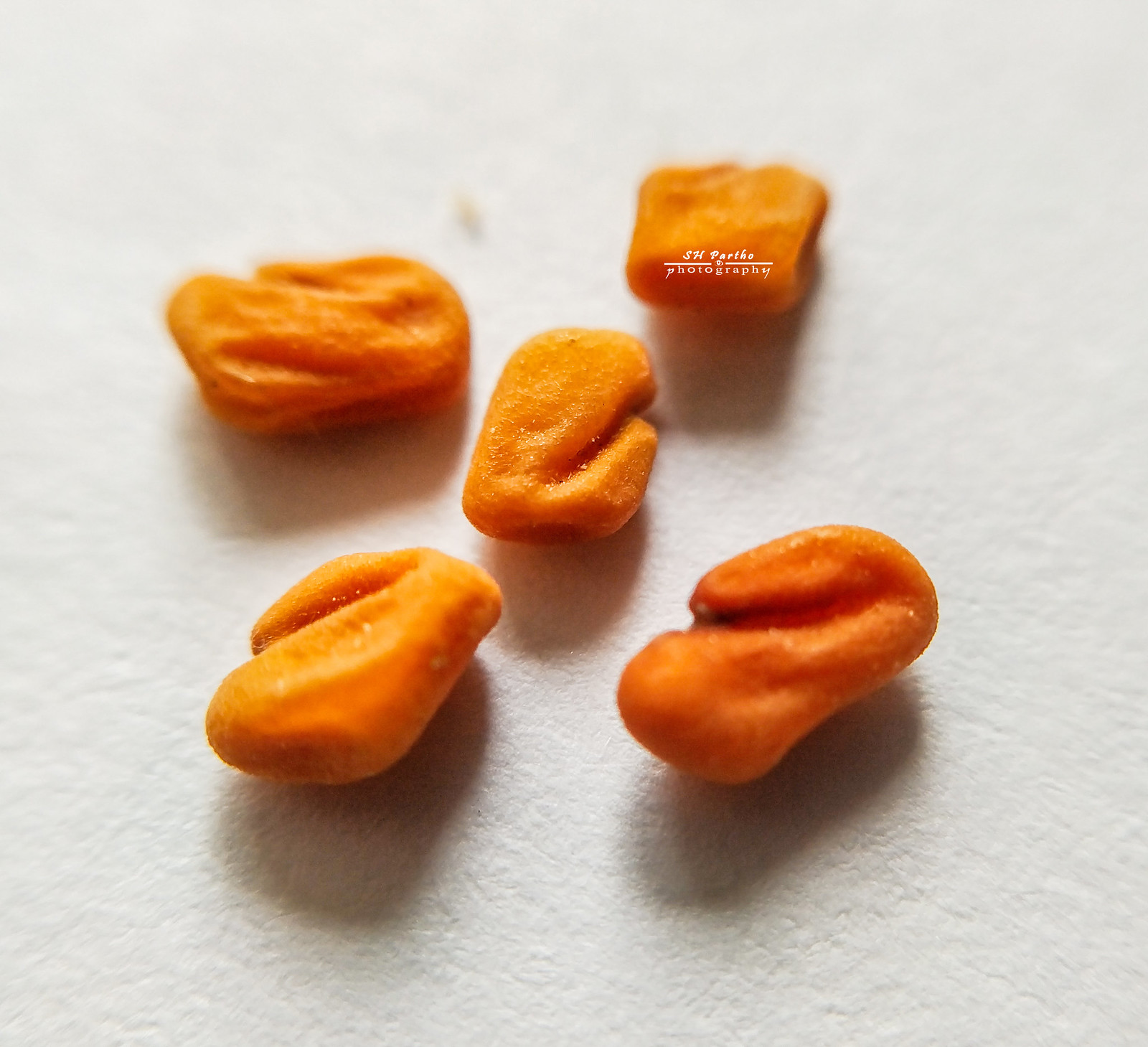The image features a large, square area with a white, granulated background, resembling a cement-like texture. At the center, there are five orange, misshapen snacks, roughly peanut-sized. Their surfaces are irregular with sectional grooves as if the material was folded. These snacks appear puffed or baked, possibly akin to cheese crackers, and they are dusted with fine white granules, likely salt. The objects are arranged with one in the center, flanked by two above and two below it, creating a precise alignment. Shadows cast on the white background suggest a light source from above. Notably, one of the snacks on the top right bears the text "S.H. Partho" followed by "photography."